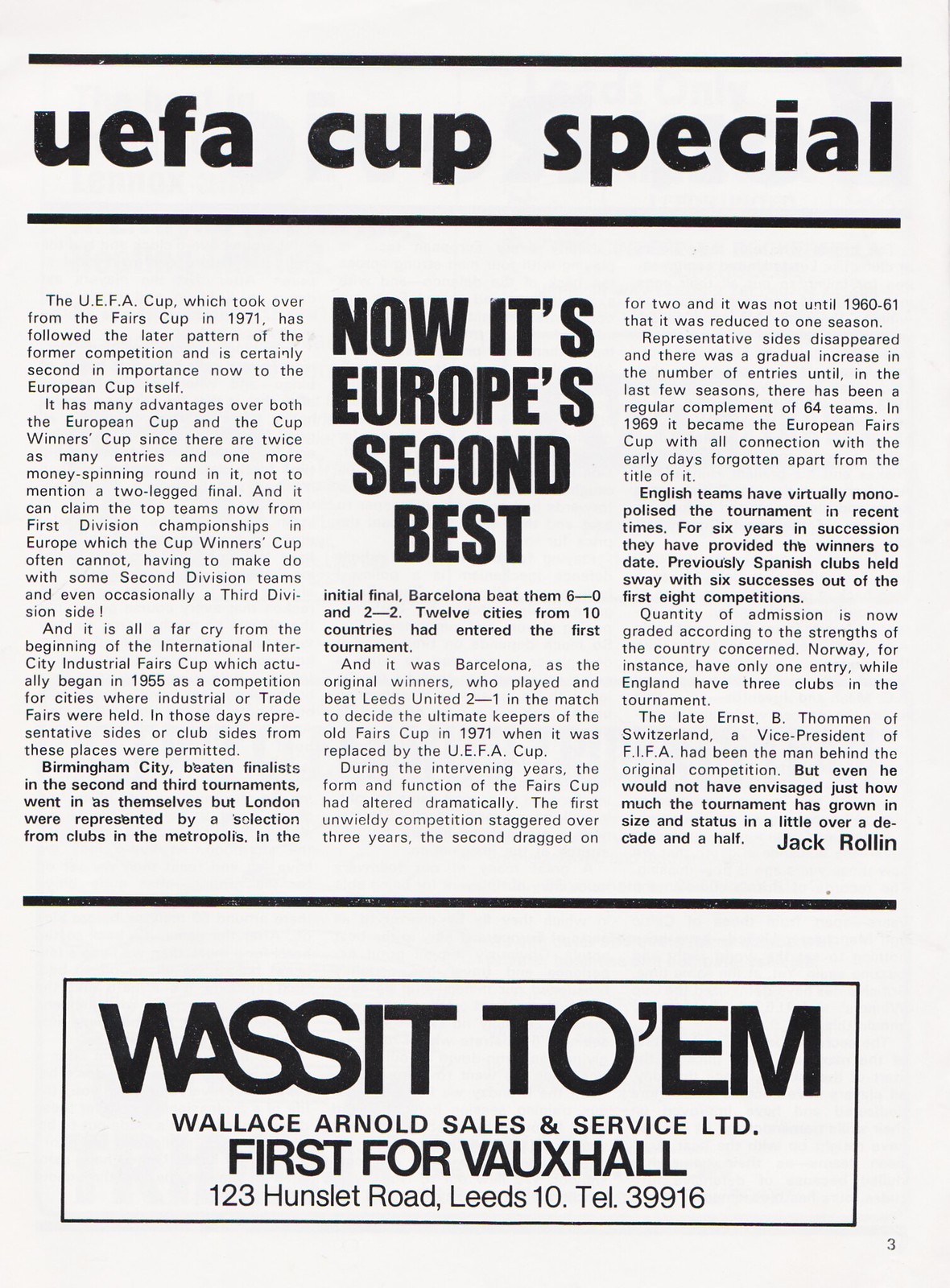This black and white newspaper clipping, page three, features a "UEFA Cup Special" header in bold black letters. Below the title, a thin black line separates the header from the main content, partitioned into three columns. The middle column is noteworthy for its bold heading, "Now it's Europe's second best." The text elaborates on the UEFA Cup, describing its evolution from the Fairs Cup in 1971 and its significance as Europe's second most prestigious club competition after the European Cup.

The left and right columns provide more in-depth history and detail about key games in the tournament. At the bottom of the page, a black-outlined rectangle houses an advertisement. In bold letters, it reads “Wassit Tuam” (a phonetic misspelling of "Watson, two M"). Beneath this, smaller text lists "Wallace Arnold Sales and Service, LTD," followed by "First for Vauxhall," and gives their address, "123 Hunslet Road, Leeds 10," along with their telephone number, "tel. 39916." The entire layout is set against a pale blue background, making the text and details stand out clearly.